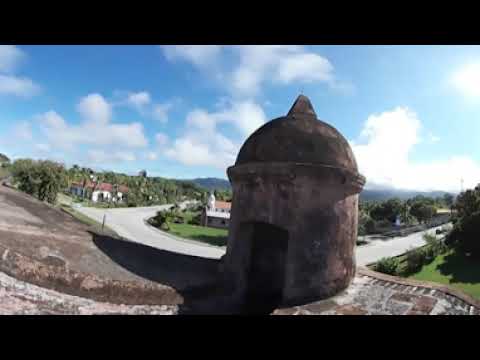In this photo, a very old and weathered cement building with a distinctive dome, topped with a pyramid-like structure, stands prominently. The dome is characterized by its gray and black coloration, hinting at its age and the natural materials used in its construction. The structure is isolated in an open lot, surrounded by varying parcels of concrete, brick, or stone paving. This lot is bordered by a network of roads that diverge in multiple directions, forming a U-shape around it. The background reveals a charming landscape with green grass, bushes, and an abundance of trees, interspersed with houses, some featuring reddish roofs. The sky is a vibrant blue adorned with wispy clouds, suggesting a sunny and clear day. The overall scene suggests a setting in a different country, exuding historical and possibly religious significance. In front of the building, a small walkway invites visitors to explore the intriguing old structure.